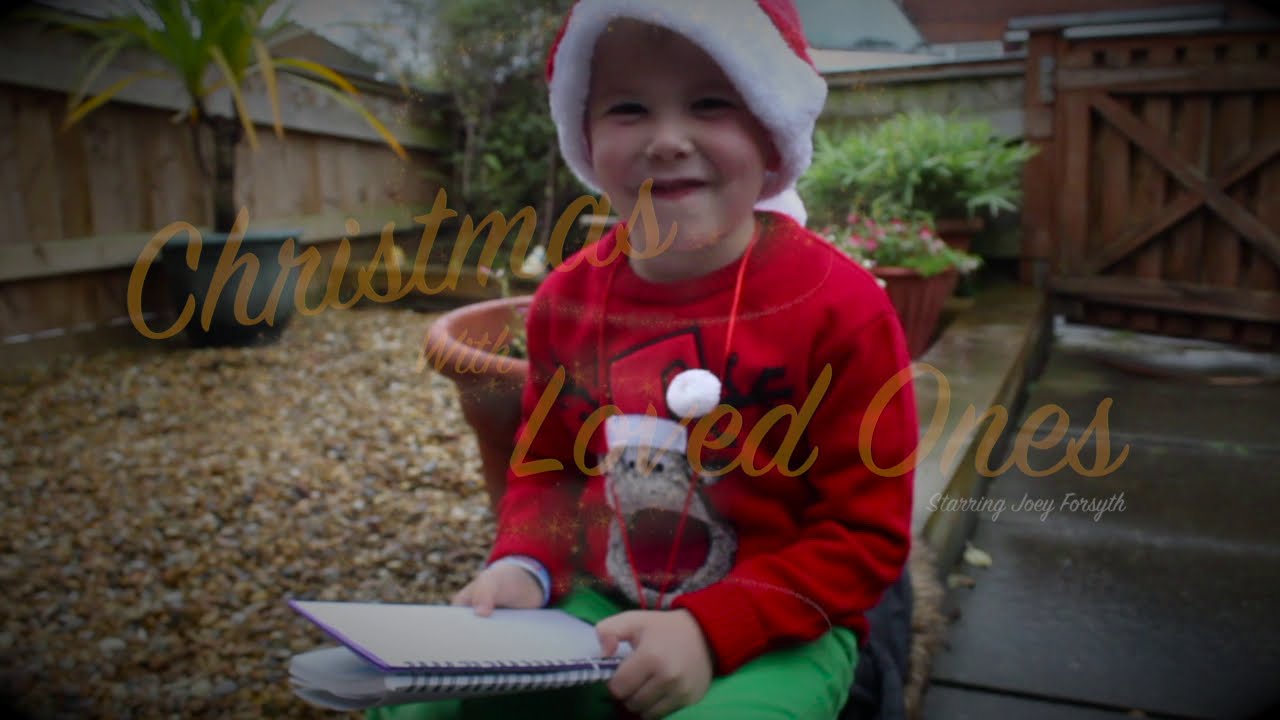In the photograph, a young, pale-complexioned Caucasian boy sits by the side of gray stairs, smiling warmly at the camera. He is wearing a festive red Santa Claus hat, a matching red long-sleeve sweater adorned with a reindeer also wearing a Santa hat, and green pants. Clutched in his hands is a purple spiral lookbook. The scene, likely taken in someone's backyard, features a large picket fence with dog-eared panels stretching from the far left to the right-hand side of the image. Behind the boy are green plants, including a large potted palm tree in a gray pot. The left side of the image shows a wooden wall with taller plants next to it, adding a natural, homely feel. At the top of the stairs on the right is a wooden door. Overlayed in faint yellow writing across the center of the photograph are the words "Christmas Loved Ones starring Joey Forsythe," suggesting this is a Christmas card or announcement.